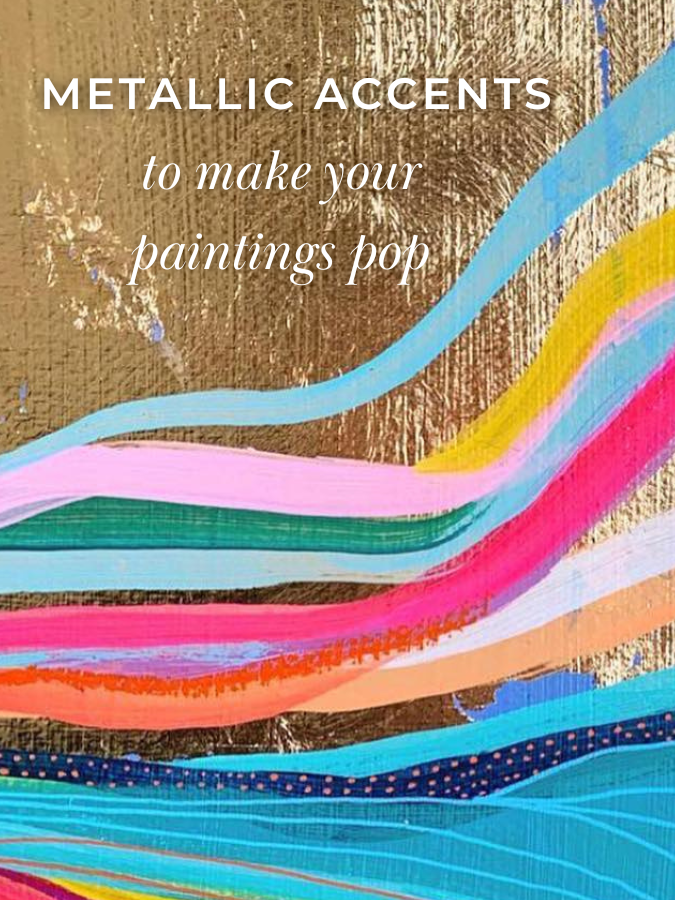The advertisement image showcases a textured, gold-brushed metallic background, with denser shading on the left and lighter on the right, giving it a subtly painted appearance. Prominently displayed at the top left, in bold uppercase letters, is the phrase "METALLIC ACCENTS," which fades into a lighter, cursive font stating "to make your paintings pop" towards the bottom, all in white. Flowing from the bottom left of the image to the top right are free-form stripes and splotches of various colors, including blue, yellow, red, teal, orange, and aqua, resembling vibrant ribbons or waves. Among these colorful streaks are playful polka dots, with a notable yellow dot near the bottom. The overall arrangement of colors and textures effectively highlights the potential of metallic accents in enhancing artistic creations.